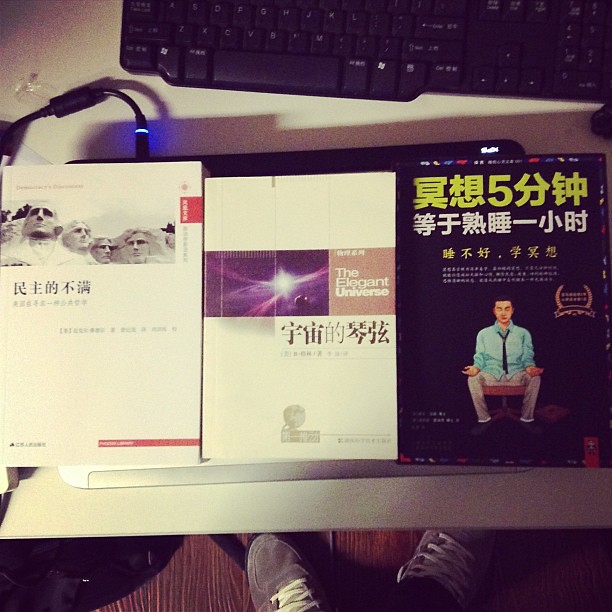This color photograph, with a sepia tone possibly due to indoor lighting, captures a detailed scene of a desk and its surroundings. The grey desk surface holds three items that appear to be either books or software program packages, each with distinct covers. The item on the left depicts Mount Rushmore and includes some Chinese characters; it is a hardcover book with a red trim. The middle item showcases a celestial image with an exploding star and the text "The Elegant Universe," also containing Chinese writing. The far-right item features a man in a blue shirt and tie, possibly sitting on a chair or toilet, with black and yellow Chinese characters at the top. A black power cord with a blue light connects to a flat black device beneath these items. The top edge of the photo shows the outline of a black computer keyboard. The photo's bottom section reveals brown floorboards, black shadows to the left, and a pair of grey sneakers with white laces on the right, suggesting someone is sitting at the desk.